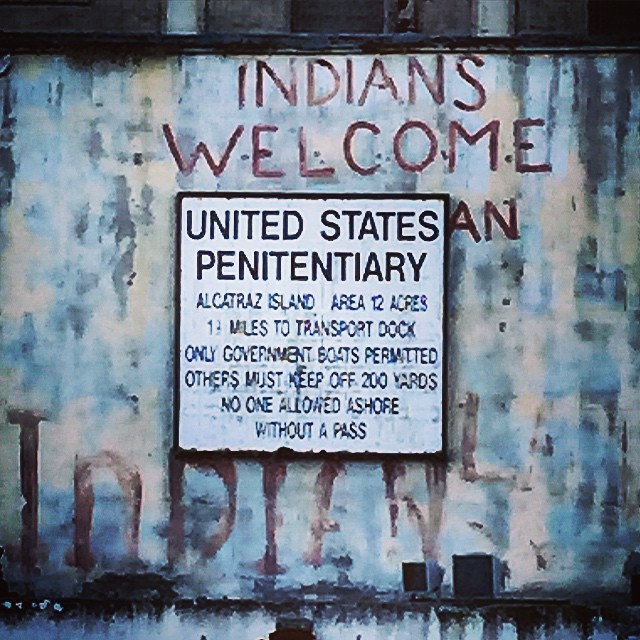The image is a photograph capturing an old, weathered wall with paint peeling off, revealing layers of white, gray, and peach hues, giving it a dirty and faded appearance. At the top of the wall, in red paint, the words "Indians Welcome" are prominently visible, albeit with some letters slightly smeared. Below this, there is an attempt at a second line of text reading "I-N-D-I-E-N," but it appears washed out and largely illegible. Centrally positioned on the wall is a rustic white sign with a black border that has begun to chip away at the edges. The sign reads in all caps, "United States Penitentiary," followed by "Alcatraz Island, Area 12 Acres" in a smaller font. It continues to list regulations: "One mile to transport dock, only government boats permitted, others must keep off 200 yards, no one allowed ashore without a pass." The entire scene conveys a sense of abandonment and historical decay.